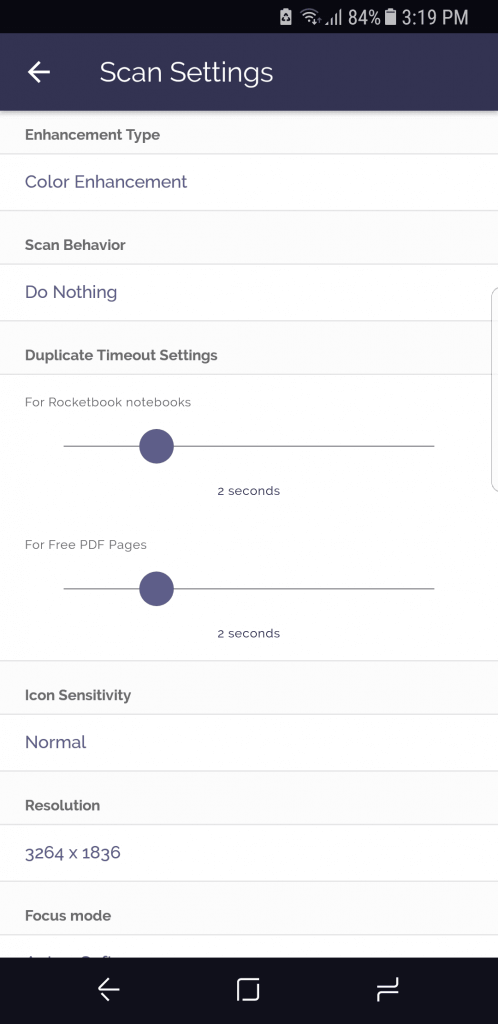The image showcases the scan settings page of a phone-based application. The settings page is structured as follows:

- **Enhancement Type**: Options for improving scan quality.
- **Color Enhancement**: Further settings to enhance colors.
- **Scan Behavior**: The current setting is "Do Nothing."
- **Duplicate Timeout Settings**: 
  - Rocketbook Notebooks: 2 seconds
  - Free PDF Files: 2 seconds
- **Icon Sensitivity**: Set to "Normal."
- **Resolution**: Set to 3264 by 1836.
- **Focus Mode**: Details are not visible; however, additional options are available if the screen is scrolled down.

The image captures only a portion of the available scan settings as there are more options below the visible section. Additionally, the:
- **Battery Life**: Displayed at the top of the screen, currently at 84%.
- **Signal Strength and Wi-Fi Status**: Indicated at the top.
- **Current Time**: 3:19 p.m.